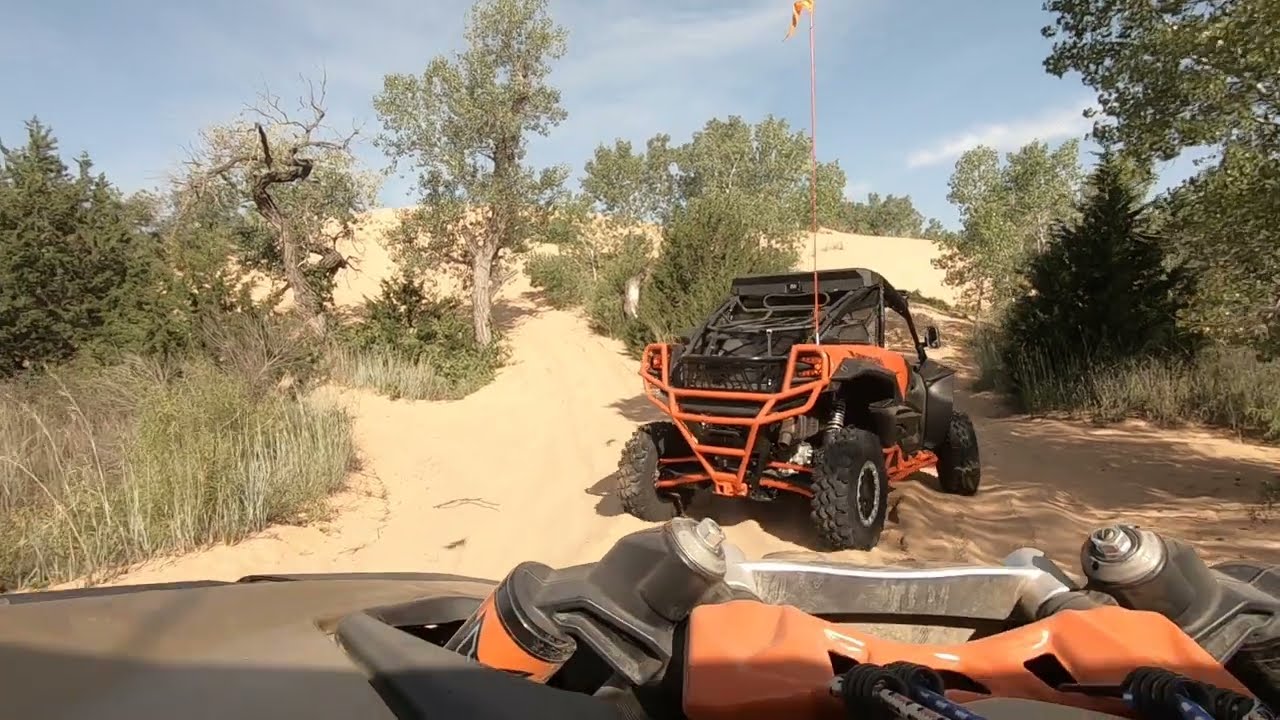The image depicts an off-road recreational adventure involving rugged four-wheeled vehicles, likely ATVs or dune buggies, navigating a dirt path through a desert landscape. Dominating the frame is a prominent black and orange vehicle at the forefront, moving away from the photographer, who's likely capturing the scene from another similar vehicle. The striking details include the orange metal frames and a tall flag mounted on the rear of the lead vehicle. Both vehicles and the dashboard of the trailing one are accentuated by the intense midday sun, illuminating the sandy terrain flanked by desert shrubs and trees on either side. The bright daylight casts clear shadows on the ground, enhancing the arid, open expanse of the backdrop. The scene lacks human figures but vividly encapsulates the essence of a sunny, adventurous off-road excursion.